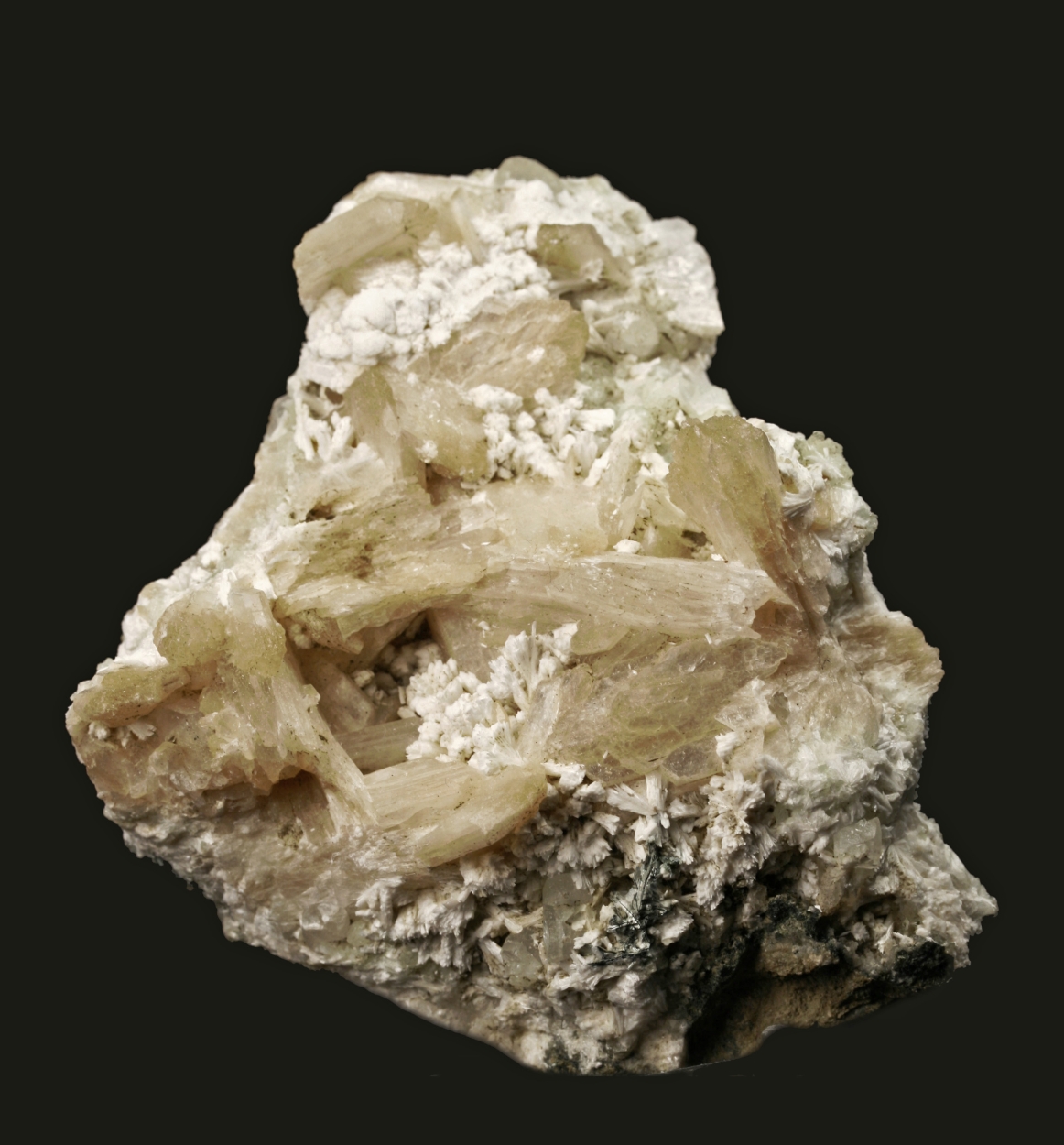This photograph is a highly detailed, up-close image of a mineral rock set against a completely black background, making the rock the sole focus of the shot. The rock, positioned centrally, appears rough with numerous imperfections and irregular ridges, displaying a blend of colors including black, white, tan, brown, silver, and yellow. The outer surface of the rock is largely gray and rough, but the interior reveals a striking crystal-like substance that appears somewhat translucent, surrounded by white, flower-like formations, which are likely hard minerals and not biological elements. The light source illuminates the rock evenly, enhancing the contrast between the crystalline core and the surrounding white mineral formations, which resemble salt compounds. The photograph provides clear detail of the rock’s texture and structure, offering a glimpse into the complex and intricate beauty of this natural specimen.